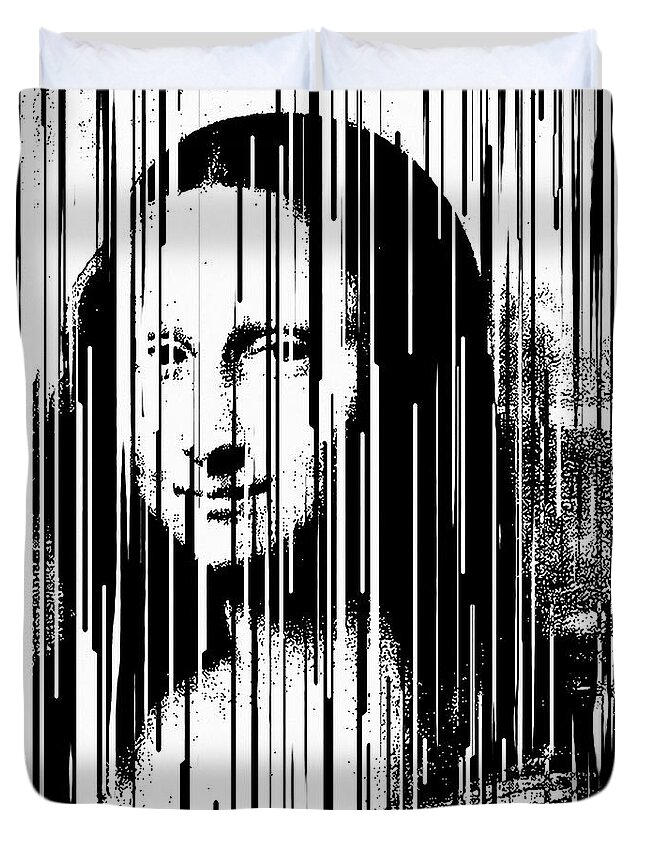The image depicts a comforter featuring a black and white rendition of the Mona Lisa. The iconic portrait, known for the woman's enigmatic smile and long black hair, has been artistically transformed with crisp, vertical lines cutting through it, creating a barcode-like effect. This graphical treatment distorts the familiar image, giving it a posterized, half-toned texture that juxtaposes light and dark intensities. The comforter's design appears layered, with the Mona Lisa image prominently displayed on the front, while two white pillows and a white mattress pad peek out from beneath, suggesting a composed and modern bedroom setting.